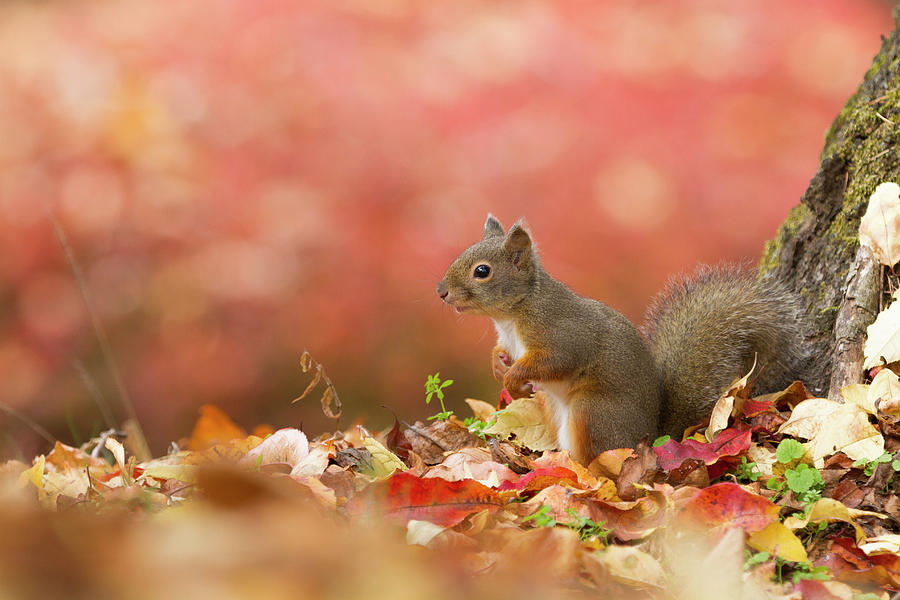This detailed photo captures the charming profile of a small gray and brown squirrel standing on its hind legs amidst a picturesque autumn setting. The squirrel, with its white belly and dark black eyes, strikes a pose with its long, bushy, curled tail held high, while its front paws are gently curled. Positioned centrally, the squirrel is backdropped by a mossy tree stump or rock, which enhances the natural setting. The ground beneath it is scattered with vibrant autumn leaves in shades of yellow, red, and brown, interspersed with a few green weedy plants and grass reeds. The photograph’s background is artistically blurred, featuring a blend of pink, orange, yellow, and green hues, ensuring that the squirrel remains the sharp focal point of this tranquil fall scene.